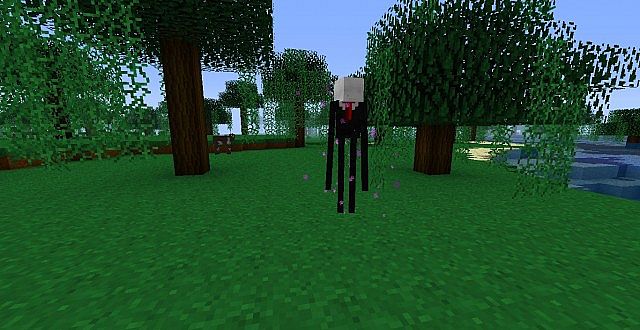A vibrant video game scene likely inspired by Minecraft, showcasing a lush green field dotted with pixelated trees. The trees feature dark, rectangular wooden trunks and cubic green leaves, set against a perfectly clear, light blue sky. On the right side of the image, a cluster of blue cubic structures adds an intriguing touch. Dominating the center is a distinctive character assembled from various prisms and blocks. This character is dressed in black, with notably long arms and legs, a striking red tie, and a gray cubic head, capturing the essence of the blocky aesthetic that defines the game.